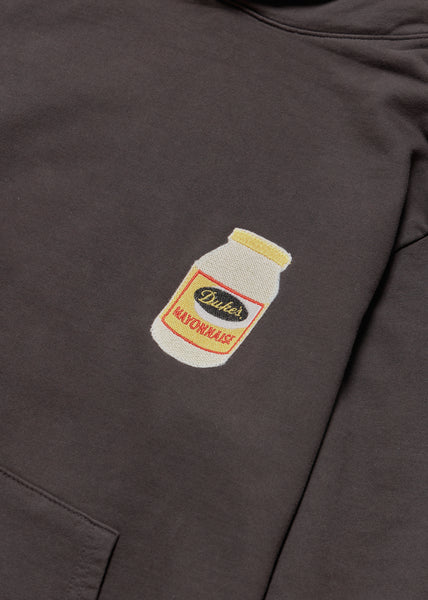This image is a close-up of the front breast area of a hoodie. The hoodie is a very dark gray, almost dark greenish gray color. On the bottom left corner, we can see the front pocket designed for hand placement and carrying small items. Detailed stitching is visible around the neck and along the shoulder and sleeve on the right side. Notably, there is a distinctive logo on the left chest area of the hoodie, depicting a jar of Duke's Mayonnaise. The jar is white with a yellow lid and label. The logo features an oval label with a black background, where the word "Duke's" is written in yellow, and "Mayonnaise" below it in red, framed with a red outline. The image highlights the detailed stitched decoration on the hoodie.